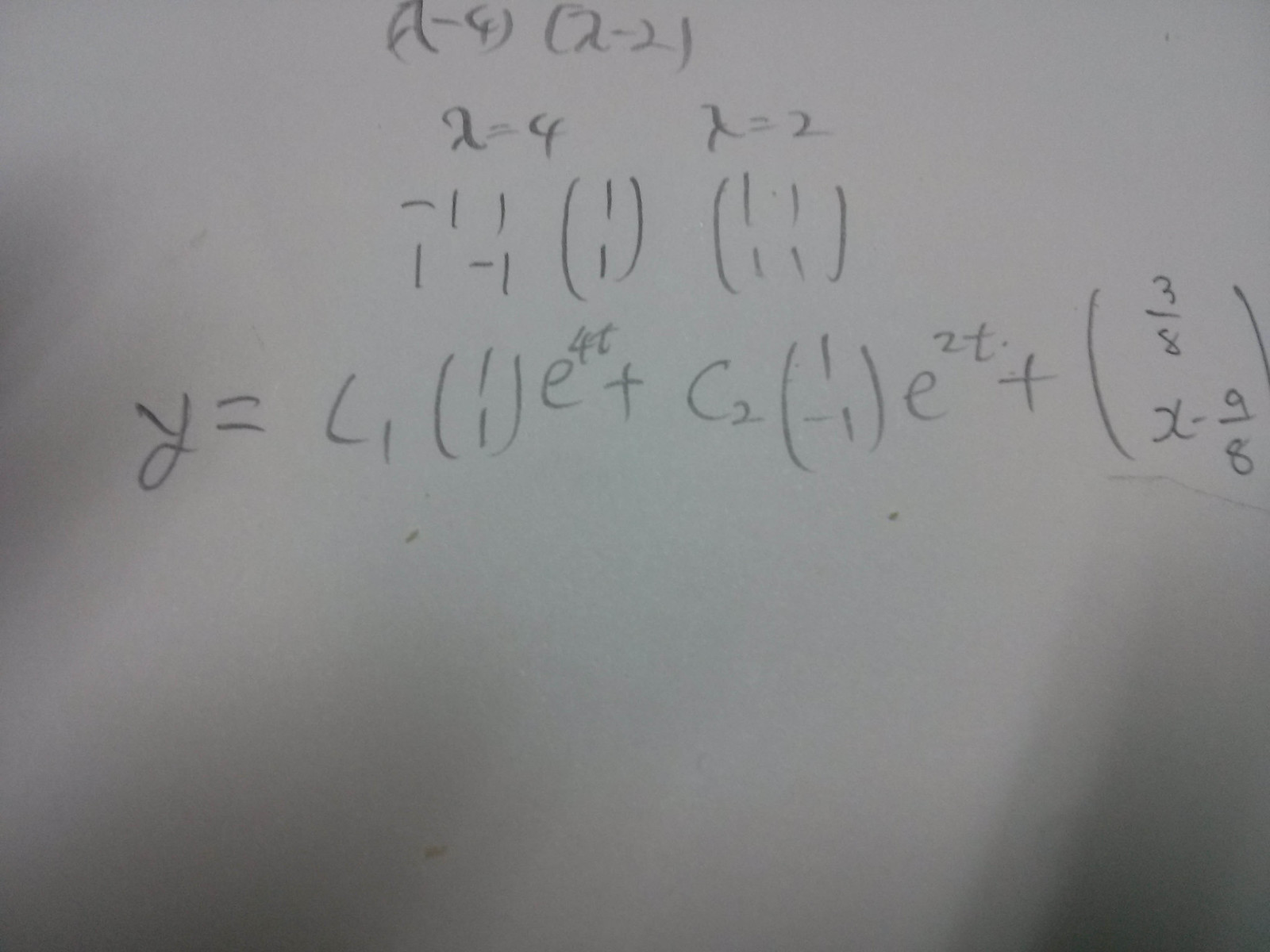The image captures a piece of paper displaying someone's math homework. The work appears to have been completed using a pencil, giving it a handwritten and slightly messy appearance. At the top of the page, the equation reads "(X - 4)(2X - 2)". Below this equation, there are additional calculations written in somewhat disorganized and difficult-to-read handwriting. One of the calculations includes "2 = 4" and "X = 2", suggesting an attempt to solve the equation. The rest of the page contains various numbers and mathematical symbols scattered throughout, contributing to a cluttered and chaotic look that reflects the challenges of working through complex math problems.